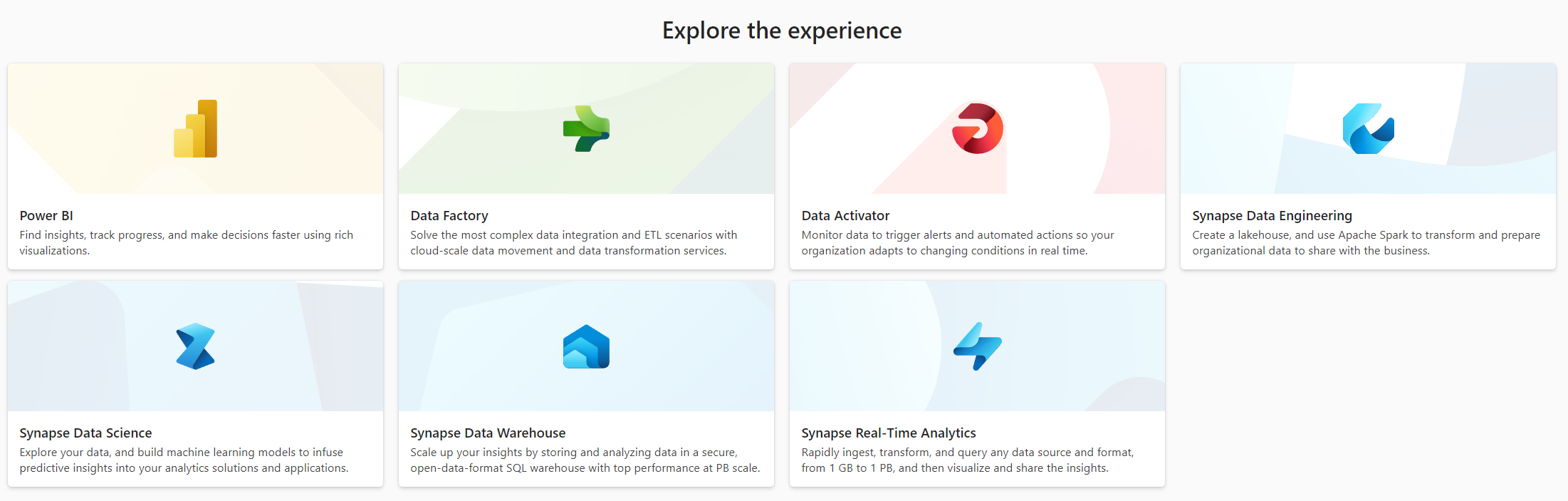This is a screenshot from an unknown web page titled "Explore the Experience." The layout is organized into two rows of sections, each describing different services. 

In the top row, from left to right:
1. **Power BI**: Find insights, track progress, and make decisions faster using rich visualizations.
2. **Data Factory**: Solve the most complex data integration and ETL (Extract, Transform, Load) scenarios with cloud-scale data movement and data transformation services.
3. **Data Activator**: Monitor data to trigger alerts and automated actions, enabling your organization to adapt to changing conditions in real-time.
4. **Synapse Data Engineering**: Create a lakehouse and use Apache Spark to transform and prepare organizational data for business sharing.

In the bottom row, from left to right:
1. **Synapse Data Science**: Explore your data and build machine learning models to embed predictive insights into your analytics solutions and applications.
2. **Synapse Data Warehouse**: Scale up your insights by storing and analyzing data in a secure, open-format SQL warehouse with top performance at petabyte (PB) scale.
3. **Synapse Real-Time Analytics**: Rapidly ingest, transform, and query any data source and format from 1 GB to 1 PB, then visualize and share the insights.